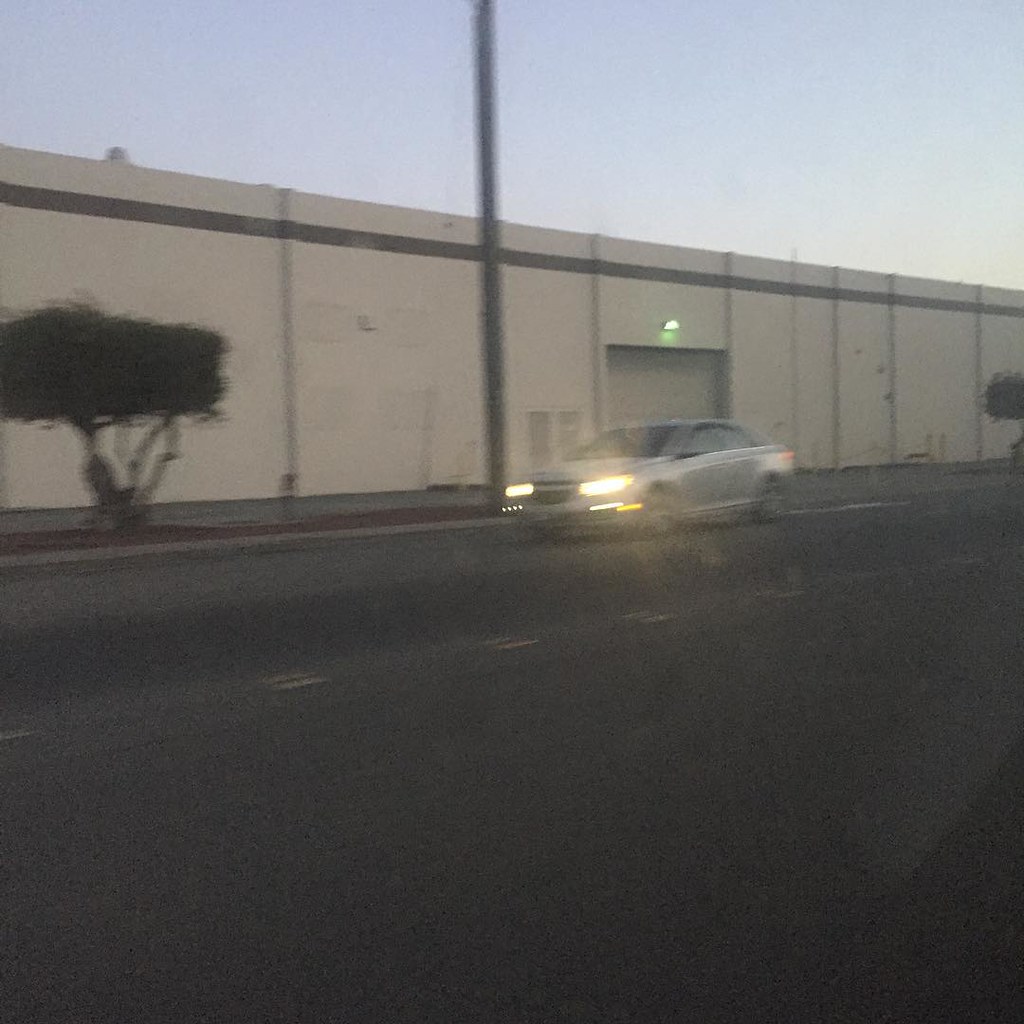In this image taken at either early morning or dusk, a silver four-door sedan travels left along a street with its headlights on, suggesting low light conditions. The backdrop features a large, tan industrial building with a prominent roll-up garage door illuminated by a light above it, implying it may be a warehouse. The building also has a venting system to the side of the garage door and a green stripe just below its roofline. In the foreground, two manicured shrubs with visible bare stems below their foliage stand along the sidewalk. The area between the street and the sidewalk is covered in brown mulch within planter beds. A telephone pole is positioned to the right of the car, extending out of the image frame into a clear, pale blue sky that hints at the time being either early morning or dusk.